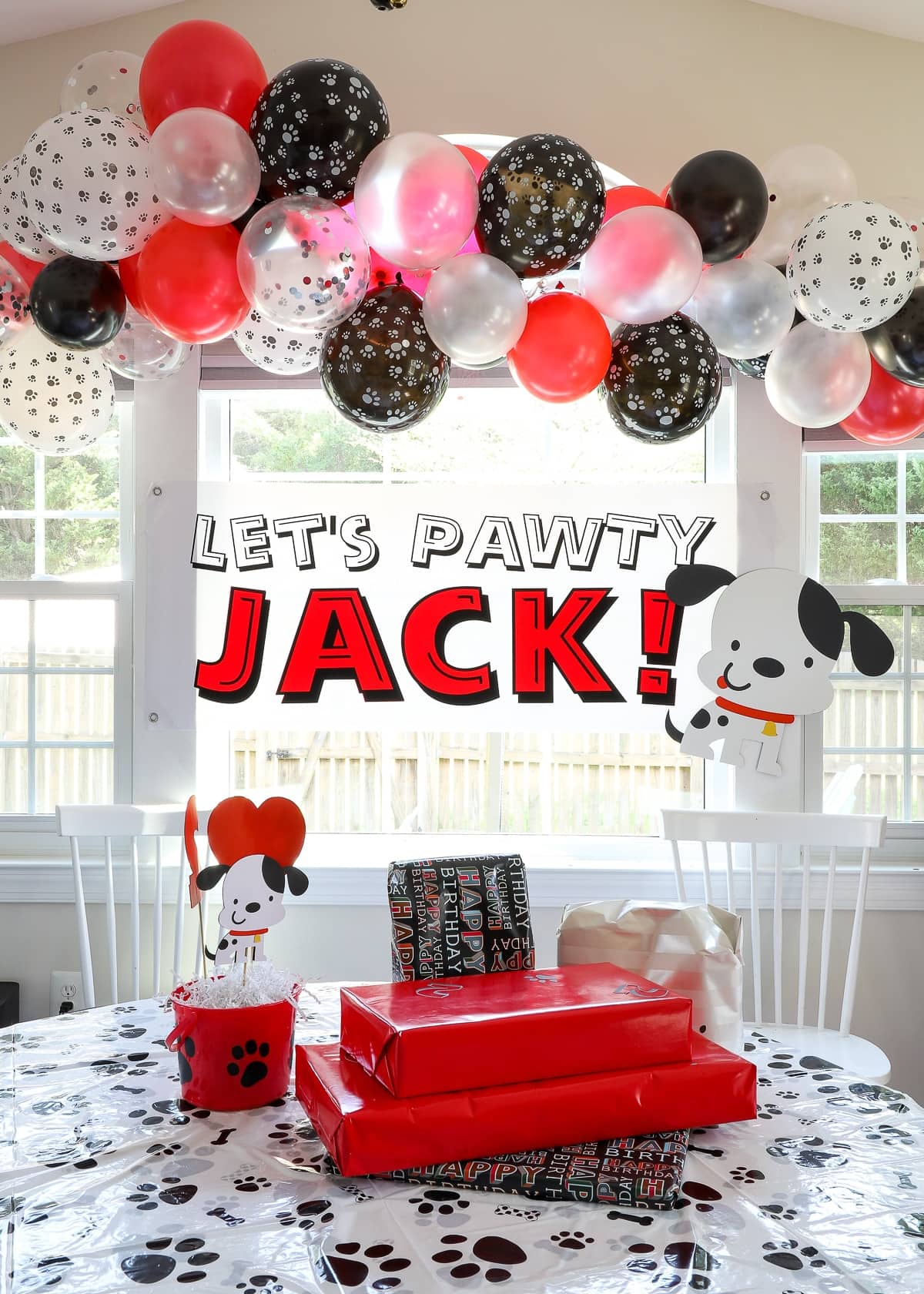The color photograph showcases a festive setup in a bright, sunny kitchen, seemingly arranged for a dog's birthday celebration. Dominating the scene is a central graphic with bold text, "Let's Paw-ty Jack!" in white and red blocky letters. Above this, a large assortment of at least two dozen balloons hangs from the ceiling, featuring a mix of red, clear, white with black paw prints, and black with white paw prints balloons. 

The room itself is bathed in natural light streaming through white-framed windows and a white doorway, revealing a sunny yard outside. The furnishings include white dining chairs with narrow dowel backs and a round kitchen table in the foreground, draped in a plastic tablecloth adorned with black paw prints. The table is laden with four or five wrapped gifts in red and black paper with "Happy Birthday" inscriptions. 

Additional decorations include a black-and-white spotted dog illustration with red hearts and a small pail featuring paw prints. Among the gifts, a tiny dog comfortably lounges in a basket, enhancing the celebratory theme. Accompanying the centerpiece text is another cutout of the black-and-white dog, adding to the cohesive dog-themed decor of the room.